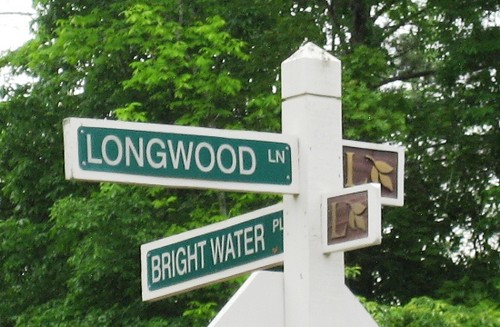In the foreground, a weathered white wooden pole with a pyramid-shaped top stands prominently. The back of a stop sign and two green street signs with white text are mounted on this thick wooden post. The signs indicate an intersection; Longwood Lane and Brightwater Place, each with a distinctive "L" and leaf design on a brown square wooden background beside them. The Longwood Lane sign faces to the left, while the Brightwater Place sign faces in a bottom-left direction. Surrounding the pole, a large green tree with numerous branches and leaves is visible, alongside an overcast grayish-white sky, faint phone lines, and a grassy area at the base of the tree. The scene captures a calm, everyday moment at a suburban-like street corner.